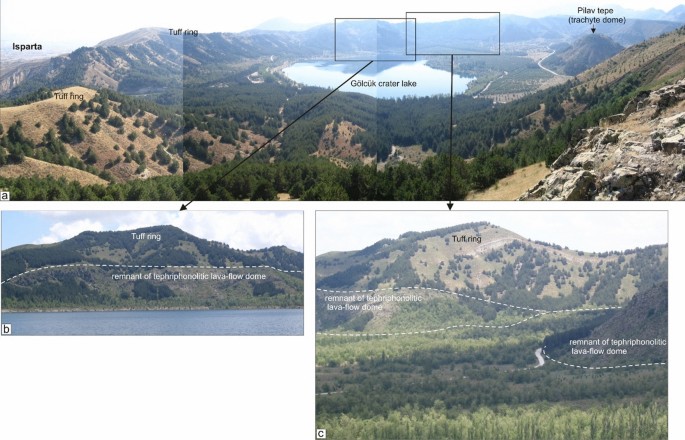The image is a detailed infographic displaying a geographical area with multiple labeled photographs overlapping one another, creating a faded effect. There are five photographs in total, each surrounded by a thin gray line.

In the upper left, there's a photograph of a brownish landscape dotted with green trees and distant mountains, labeled "Isparta." In the middle top, partially overlapping the first, is an image labeled "Tuff Ring" with a central feature identified as "Gulchuk Crater Lake." To the right of this is another photo of a large hill, annotated with "Pleitepe" and underneath it "Trachite Dome" with a downward arrow, suggesting volcanic activity. 

The lower left corner contains a rectangular image with a white dashed line crossing it horizontally, labeled again with "Tuff Ring" and partially obscured text suggesting "remnant of a phreatomagmatic lava flow dome." Finally, the lower right corner showcases a larger rectangular photograph also labeled "Tuff Ring," with additional white print and dashed lines marking geological features.

Overall, this infographic appears to illustrate various geological formations such as craters and volcanic domes within a mountainous region, possibly using digital overlays for educational purposes.